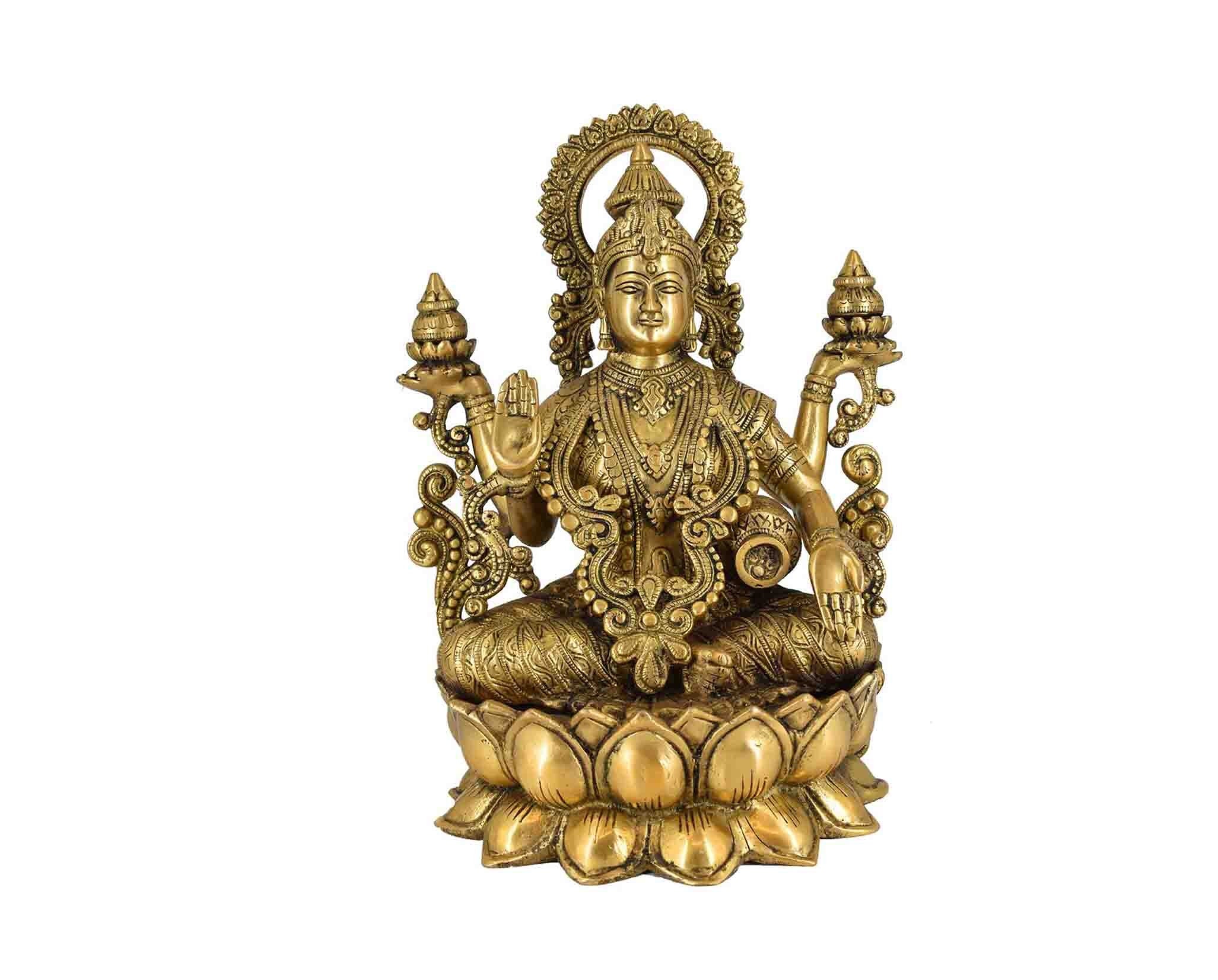This image portrays an intricately crafted brass statue of a South Asian river goddess seated on a lotus flower. The goddess, depicted as an Indian woman, is in a meditative pose with her legs crossed. She holds one hand with its palm facing downward and the other with its palm facing upward. A terracotta pot rests under one arm, adding to the symbolism of the figure. She is adorned with a large necklace that cascades down to her foot and is wearing a pointed hat with a medallion that hangs over her forehead. The lotus flower serves as a base and also forms a chair-like structure at its back, with each corner embellished by round, pointed protrusions resembling lotus buds. Additionally, there is a circular halo behind her head, completing the divine and serene representation. The statue is set against a white background, enhancing its gold and brownish hues, and features ornate details that reflect its cultural and religious significance.